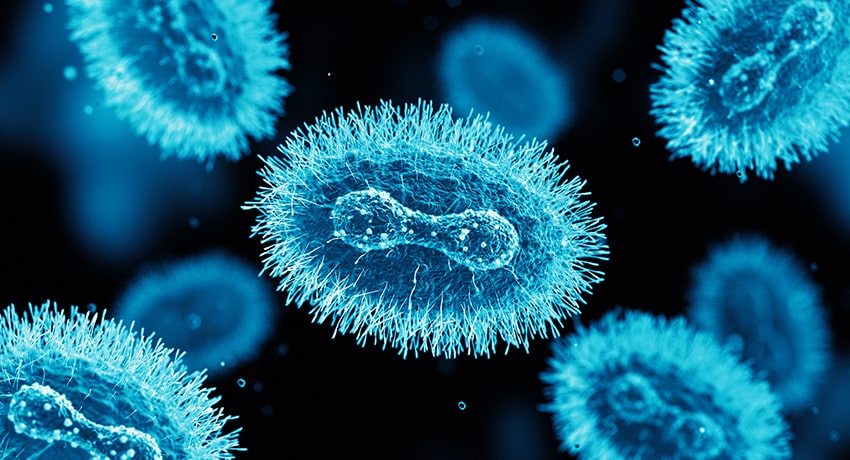This horizontally aligned rectangular image presents a detailed microscopic view of monkeypox. Dominating the frame is a sharply focused, oval-shaped blue structure at the center, surrounded by a solid black background. This central cell features a distinctive dumbbell-shaped formation, adorned with small white nodules. The surface of the cell is enveloped by a crisscross pattern of fine, hair-like filaments.

Surrounding this central structure are several additional oval-shaped cells in the corners of the image. The cell in the lower left is partially visible and slightly in focus, while those in the upper left, upper right, and lower right corners are more blurred. Multiple other cells, all equally blurred, float both above and below the central cell, adding depth to the black expanse. The overall visual effect is reminiscent of a cluster of dividing cells, with each exhibiting a characteristic blue hue and a transparent quality.